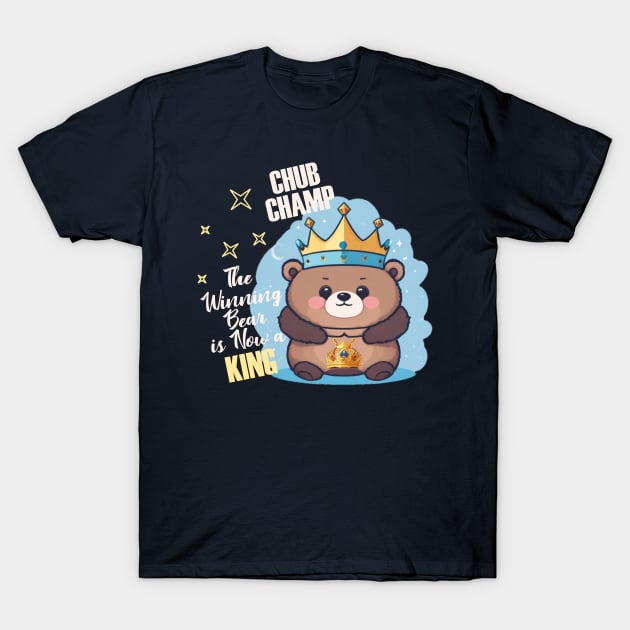This photograph showcases a black short-sleeve t-shirt set against a plain grey backdrop. Dominating the center of the shirt is a vibrant, cartoonish illustration of a brown bear with stylized pink cheeks. Adorning the bear's head is a golden crown with a blue band and gem embellishments, while the bear is holding a more realistic crown against its tummy. Surrounding the bear is a light blue outline that includes a moon and stars to emphasize the celebratory nature of the scene. Above the bear, in bold letters, it reads "Chub Champ." To the left of the bear, in cursive text, it says, "The winning bear is now a king," with the word "king" highlighted in yellow. Completing the design, stars are scattered around the text, adding to the momentous occasion being depicted.